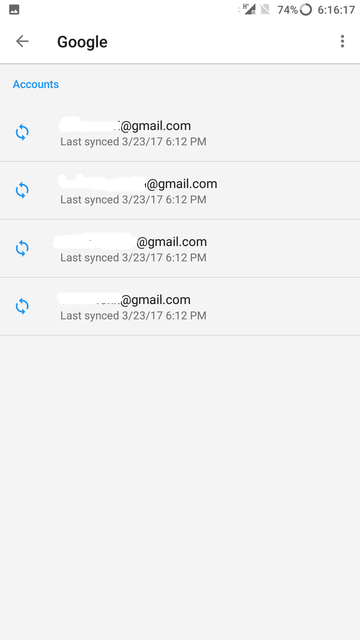The screenshot shows a smartphone screen with a time display of 6:16 and 17 seconds, as well as a battery indicator showing 74% battery life. The screen appears to be displaying Google account synchronization details. The Gmail addresses are partially obscured for privacy. Below are the details:

1. The first account was last synced at 6:12 PM on the 23rd.
2. The second account was also last synced at 6:12 PM on the 23rd.
3. The third account followed the same pattern, syncing at 6:12 PM on the 23rd.
4. The fourth account was synced at the same time, 6:12 PM on the 23rd.

All four Gmail accounts were synchronized simultaneously. The interface includes a "Refresh" button with a blue arrow icon, which can be used to update the sync status. 

The text is displayed in white on a dark gray background, with the synchronization timestamps in lighter gray. The partially visible Gmail addresses are in black text on a grayish background. Blue accents highlight interactive elements like accounts and arrows, ensuring crucial details are visually distinct amidst the overall grayscale theme.